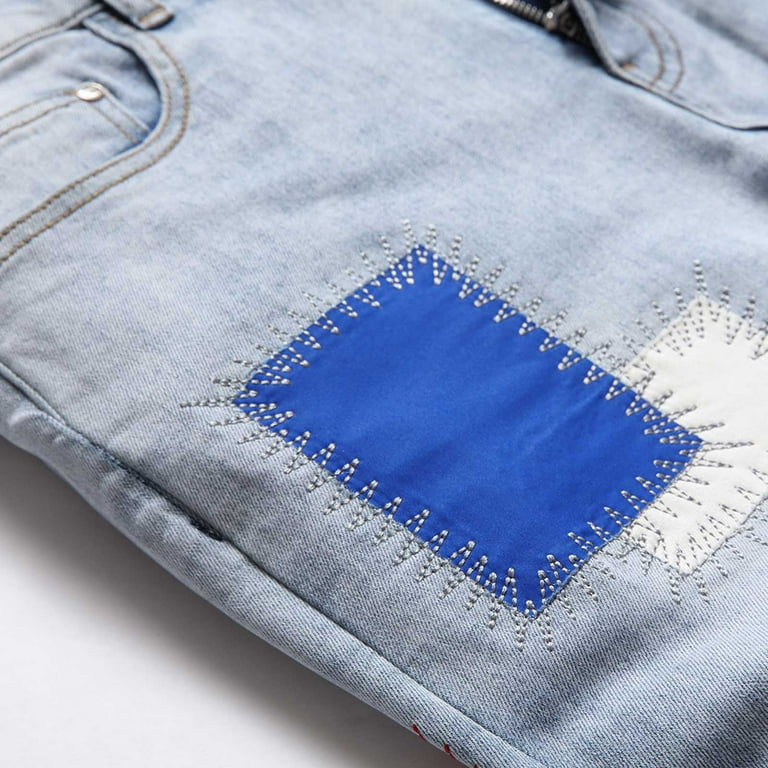The close-up vertical rectangular image showcases a pair of light, acid-washed jeans laying on a white surface. The focal point is the upper section of the right pant leg, just below the pocket and well above the knee. These jeans are older and slightly faded, but in good condition. Highlighted prominently on the right thigh area are two decorative patches: a larger vertical blue rectangle and, partially tucked underneath it, a smaller horizontal white rectangle. Both patches are intricately sewn on with distinctive zigzag (possibly whip stitch) white or silver stitches radiating from the edges, giving a 'ray of light' effect. The pocket is visible in the upper left of the image, while the lower right corner shows part of the fly and crotch area.